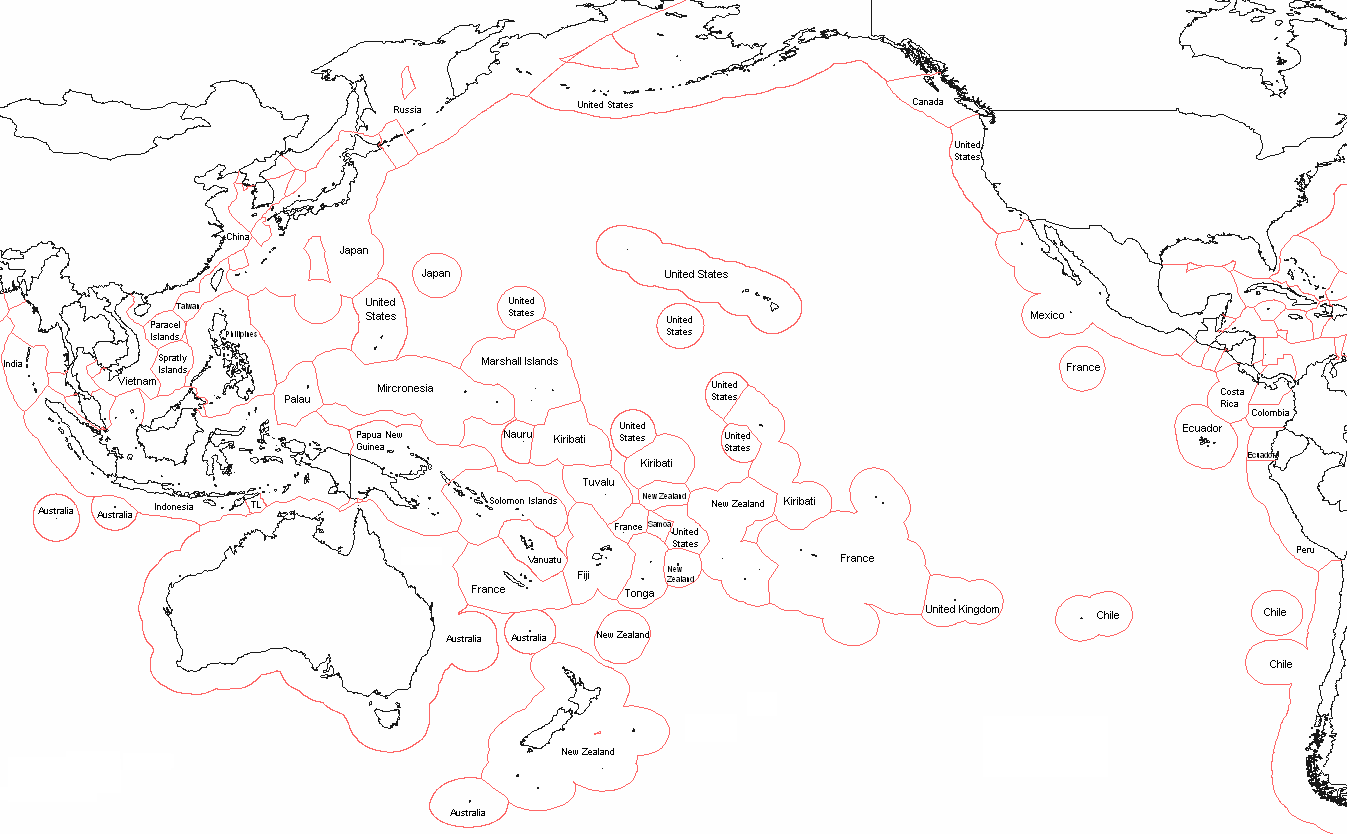This image features a predominantly white background with a world map outlined in black at its center. Various countries are singled out by red circles; notable among these are the United States, France, New Zealand, and the United Kingdom. Additionally, smaller red marks trace the map's borders and scatter along the top edge, giving a sense of additional emphasis or focus. To the right of the main map, there is a smaller inset map of the United States, also accented with similar red markings. The entire arrangement feels peculiar due to the seemingly random yet purposeful placement of these red circles and highlights.